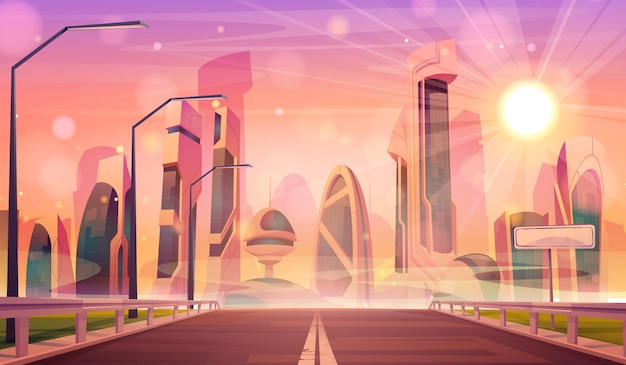This detailed depiction showcases an AI-generated, futuristic cityscape seen from a dark, guarded roadway leading into the city. The scene is awash with a surreal blend of hues, dominated by an orange tint cast by a large, round sun perched in the upper right corner of the sky. The sky itself graduates from a deep violet at the top to varying shades of peach as it descends. The street is lined with sleek, modern street lamps featuring flat light panels instead of bulbs. 

The architectural marvels standing tall against this vibrant backdrop are a mix of white, ultra-modern buildings, their sleek designs accented by stark black windows. Some structures are tall and thin, while others are cylindrical, and still others are circular, all contributing to the futuristic ambience. The solitary visible sign bears no writing, emphasizing the scene's minimalist aesthetic. The road, painted with a double line in the center, appears slightly orange-tinted, reflecting the warm glow of the sun. Notably, the entire city is devoid of people, adding an eerie, tranquil feel to this clean and brightly colored urban vision.